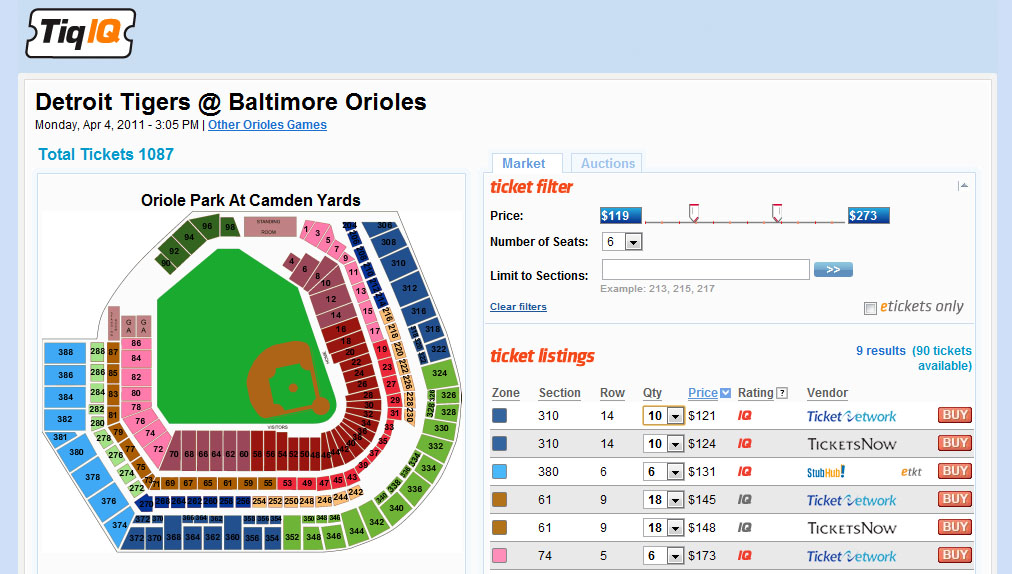A detailed map of available tickets for a baseball game is shown on the TICIQ website. The website logo "TIQ" is in black and "IQ" is in orange, displayed at the top part of the image with a gray box underneath it. Inside the gray box, in black text, it reads "Detroit Tigers at Baltimore Orioles" with the game date and time listed as Monday, APR 4-2011 at 3:05 p.m. Below, in blue text, are options for viewing other Orioles games and the total number of available tickets, which is 1,087.

The image features a seating chart for Oriole Park at Camden Yards. The baseball field is depicted in green, surrounded by brown areas representing the infield. The first set of rows around the field is color-coded in reddish and pink hues. As the sections extend outward, the colors transition from pink and red to brown, blue, orange, and back to various shades of blue and green, indicating different pricing or availability zones. 

On the right-hand side, there's a user interface with various tabs labeled "Market" in blue, and "Auction." Under "Market" in orange, there is a ticket filter feature showing prices ranging from $119 to $173, with options to select the number of seats, limit to specific sections, and view ticket listings. Each listed ticket provides detailed information including different zone colors, section numbers, row numbers, quantities, prices, brands, and vendors.